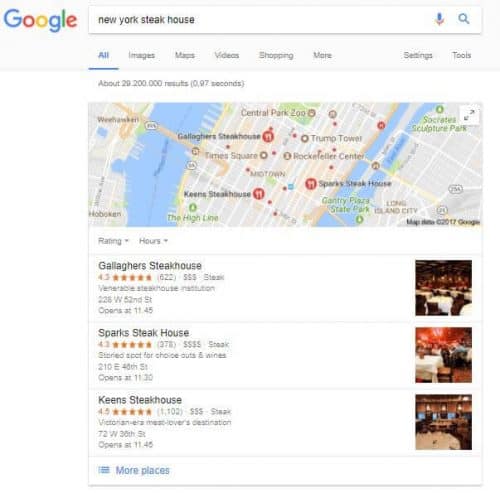The image is a detailed screenshot of a search result page. At the top, the word "Google" is spelled out in colorful letters: blue, red, yellow, blue, green, and red respectively. Below the logo is a search box, outlined in gray with a white background. In the search box, "New York Steakhouse" is typed in black. To the right of the search box, there is a blue microphone icon and a blue magnifying glass. Below the search bar, there are several blue and gray text options including "All" (in blue and underlined), "Images", "Maps", "Videos", "Shopping", "More", "Settings", and "Tools".

The page has a white background displaying the text "About 29,200,000 results (0.97 seconds)" at the top. Featured prominently is a map showing parts of New York City with water bodies on both sides and several landmasses. The map highlights locations like Keens Steakhouse, Gallagher's Steakhouse, Trump Hotel, Rockefeller Center, Times Square, Sparks Steakhouse, Gantry Plaza State Park, and The High Line.

Underneath the map, the background is white and light gray. Listed are various steakhouses with their ratings and number of reviews. Gallagher's Steakhouse has 4.3 stars from 622 votes, marked with three dollar signs. Sparks Steakhouse has 4.2 stars from 378 votes, marked with four dollar signs. Keens Steakhouse has 4.5 stars from 1,100 reviews, marked with three dollar signs. Each listing is separated by a thin gray line, and descriptions are followed by the text "Steak".